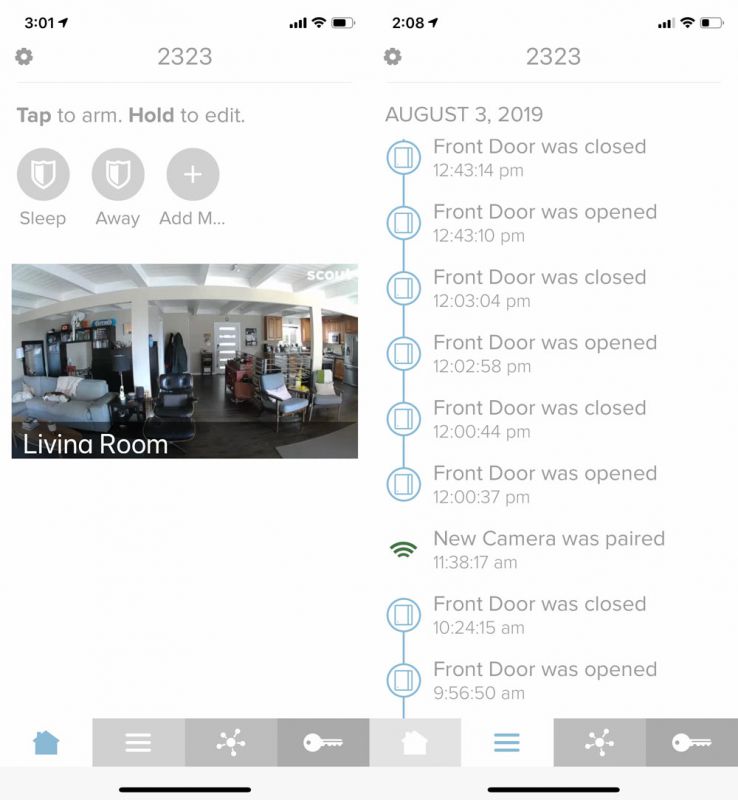The image displays two smartphone screens side by side.

On the left screen:
- In the top-left corner, the number "301" is visible.
- The top-right corner shows cellular signal bars, Wi-Fi strength, and a battery icon at approximately 50%.
- Below that, there is a Settings icon followed by the number "2322".
- The text "Tap to arm, tap and hold to edit" is prominently displayed.
- Underneath are three circular icons labeled "Sleep," "Away," and "Add...".
- A photograph is visible below these icons, depicting a living room that appears to also include a kitchen area.

On the right screen:
- The top-left corner shows the number "208".
- The top-right corner displays cellular signal bars, Wi-Fi connectivity, and a battery icon showing roughly 30%.
- There is a timestamp: "August 3rd, 2019".
- Below, a log lists activities involving the front door:
  - "Front door was closed, 12:43 PM"
  - "Front door was opened, 12:43 PM"
  - "Front door was closed, 12:43 PM"
  - Specific timestamps of door activities are detailed:
    - First event at 12:43:14 PM
    - Second event at 12:43:10 PM
    - Third event at 12:43:04 PM
  - "Front door was opened, 12:02:58 PM"
  - "Front door was closed, 12:12:44 PM"
  - "Front door was opened, 12:37 PM"

These detailed logs help in tracking the exact times the front door was opened and closed.